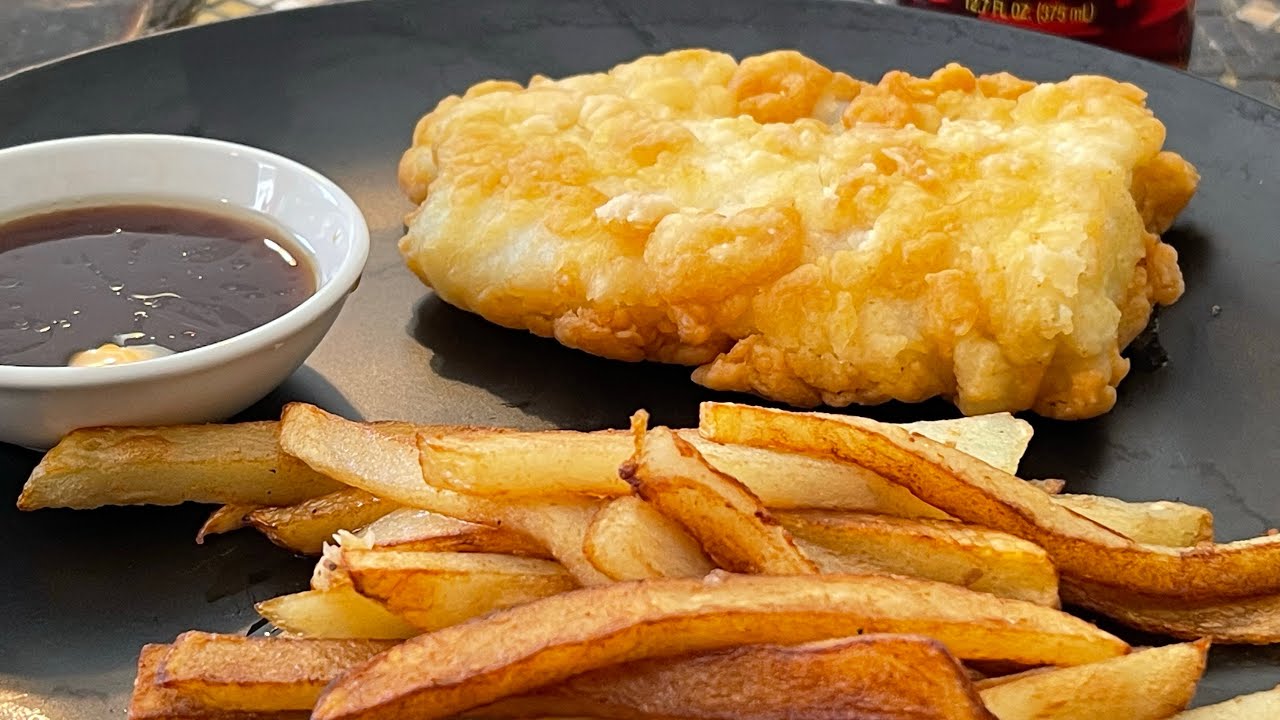This photograph showcases a meticulously-plated dish of fish and chips, presented on a round, dark gray ceramic plate. The centerpiece is a single piece of perfectly battered cod, its golden-brown crust boasting a delightful range of hues from light to slightly darker shades. Arrayed in front of the fish are French fries, varying in doneness with some being crispy and golden, while others are softer and less cooked. To the left of the plate, a small white bowl filled with malt vinegar, textured and brown, hints at the potential for tangy flavor enhancement. The scene suggests an al fresco dining experience, as evidenced by the reflective surface of the malt vinegar bowl and the blurred outdoor backdrop. No text or captions are present within this visually appealing and appetizing composition.